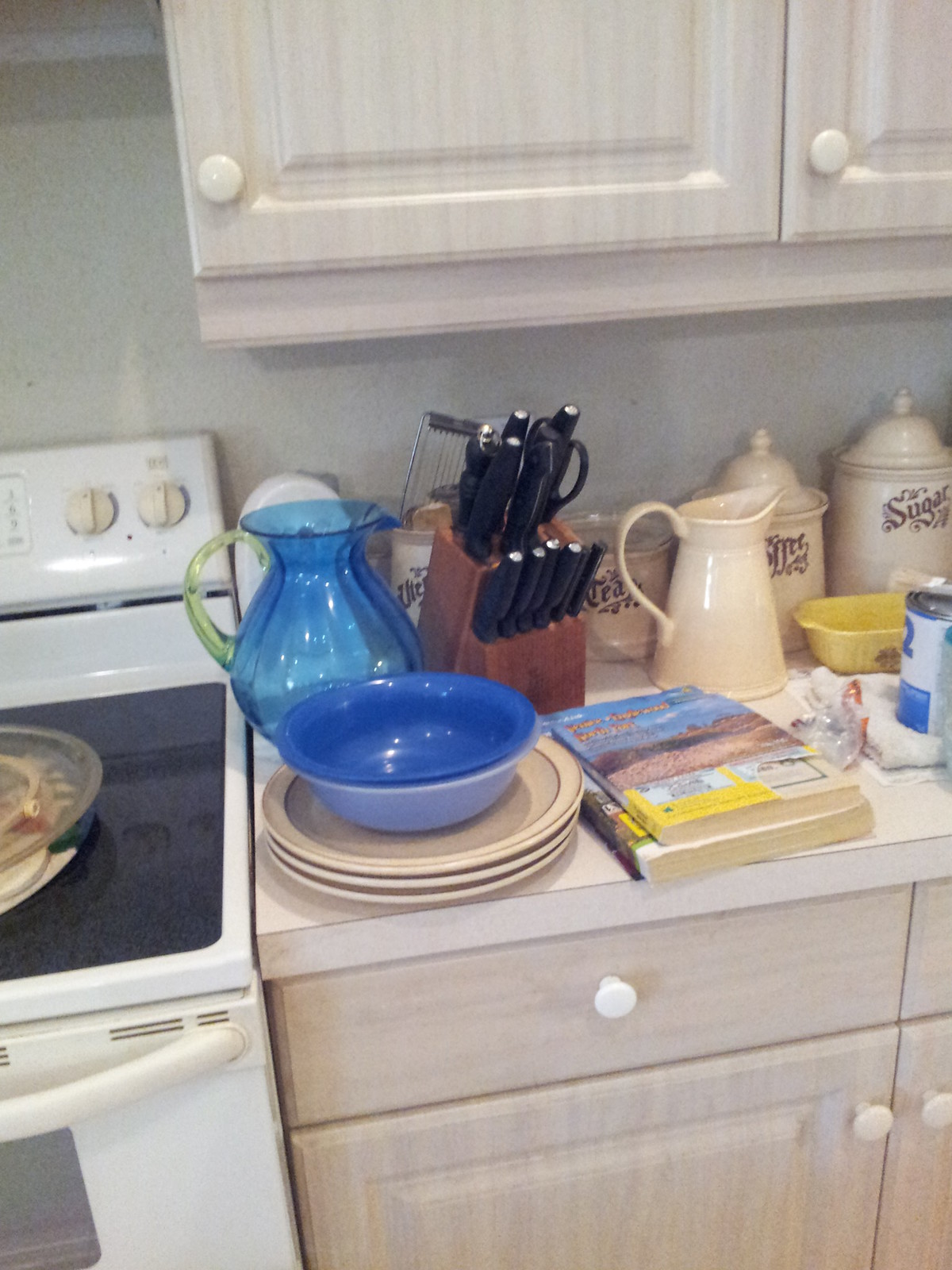The image captures a close-up section of a kitchen, focusing on a light-colored wooden cabinet with an almost cream-like hue. On top of this cabinet sit several dishes in light brown and blue hues, adding a touch of color to the scene. Nestled among the dishes, there’s a ceramic, cream-colored milk jug and a small stack of what appear to be yellow pages. A wooden knife rack is also visible, securely holding multiple knives with black handles, hinting at a well-equipped kitchen. Above the main cabinet, the upper cabinet doors can be seen. To the left of the cabinet, a portion of a stove comes into view, showcasing its oven door with a white handle and two white knobs, blending seamlessly with the kitchen's soft, neutral palette. This close-up provides a glimpse into a well-organized and serene kitchen corner.